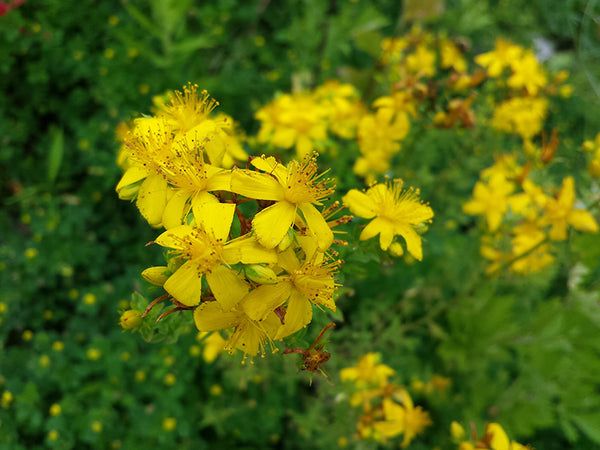The photograph captures a cluster of vividly yellow flowers against a blurred green background interspersed with subtle yellow specks. Dominating the composition, the flowers in the forefront feature five flat petals each, fully open and showcasing a vibrant yellow hue. Emerging from the center of these blooms are numerous hair-like, yellow strands that culminate in tiny reddish-brown tips resembling seeds. The flowers, grouped closely in a prominent bunch of about four to seven, also reveal nascent buds still closed underneath some of the blossoms. The background, enveloped in a green hue suggestive of surrounding vegetation or bushes, fades into a soft blur, adding depth and drawing the viewer's focus toward the finely detailed and strikingly beautiful yellow flowers.